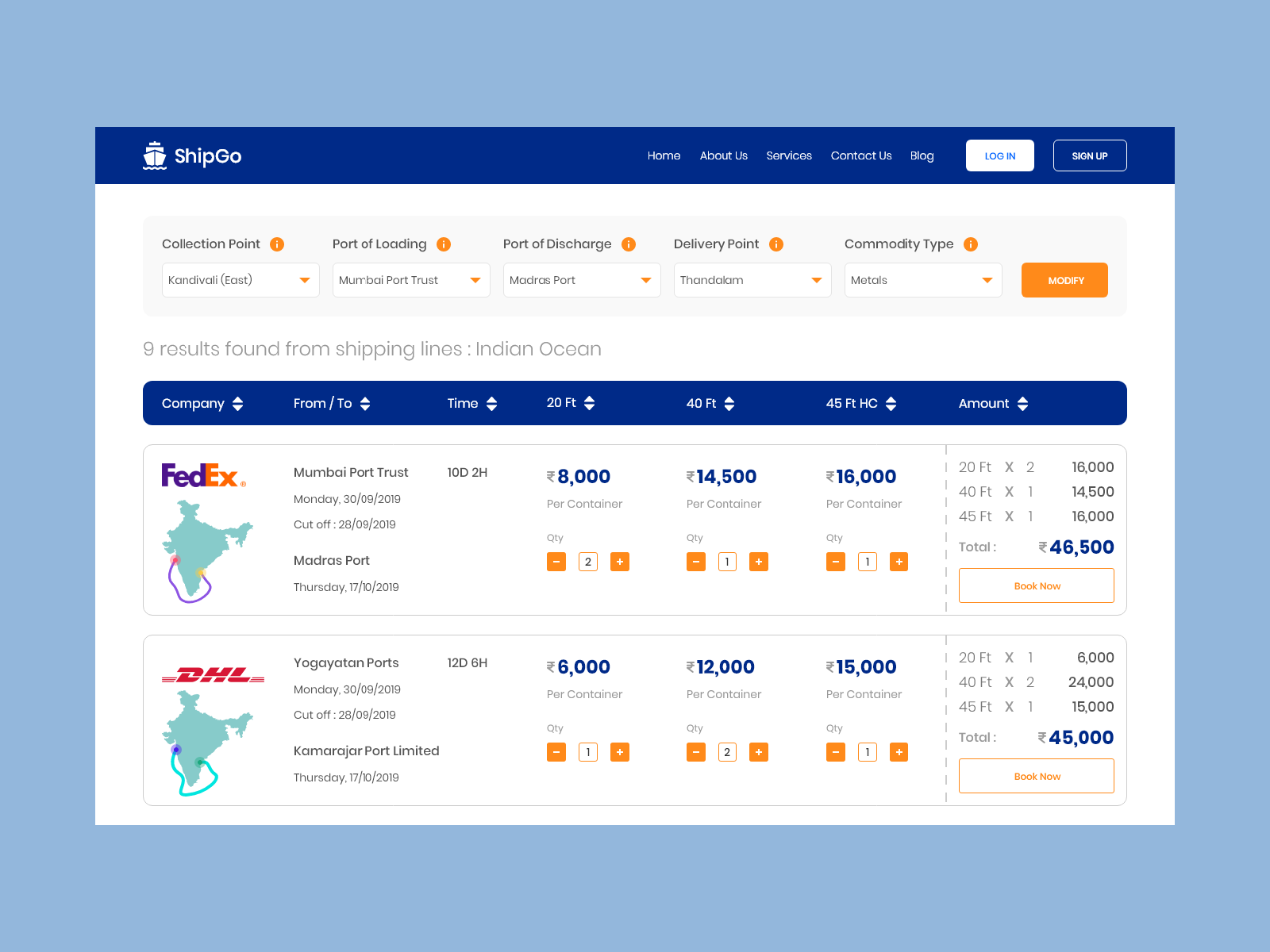The image depicts a themed shipping box placed against a light blue background. The box features a dark navy blue border at the top. In the top left corner, there's an illustration of a boat sailing head-on towards the viewer with the text "Ship Go" next to it. On the right side of the box, navigation options are listed: "Home," "About Us," "Services," "Contact Us," and "Blog." Beneath these options, there are two buttons: a white "Sign In" button and a blue "Sign Up" button.

Below this navigation bar, the text "Collection Point" appears above a drop-down menu, though the content of the menu is unclear. To its right is the label "Port of Landing" with a drop-down menu that reads "Whereby Port Trust." Another label, "Port of Discharge," appears next to a drop-down menu that shows "My Madrid, Madrid Port." The final label, "Delivery Point," is followed by an input field labeled "Datum." To the right of this field is an orange button labeled "Modify."